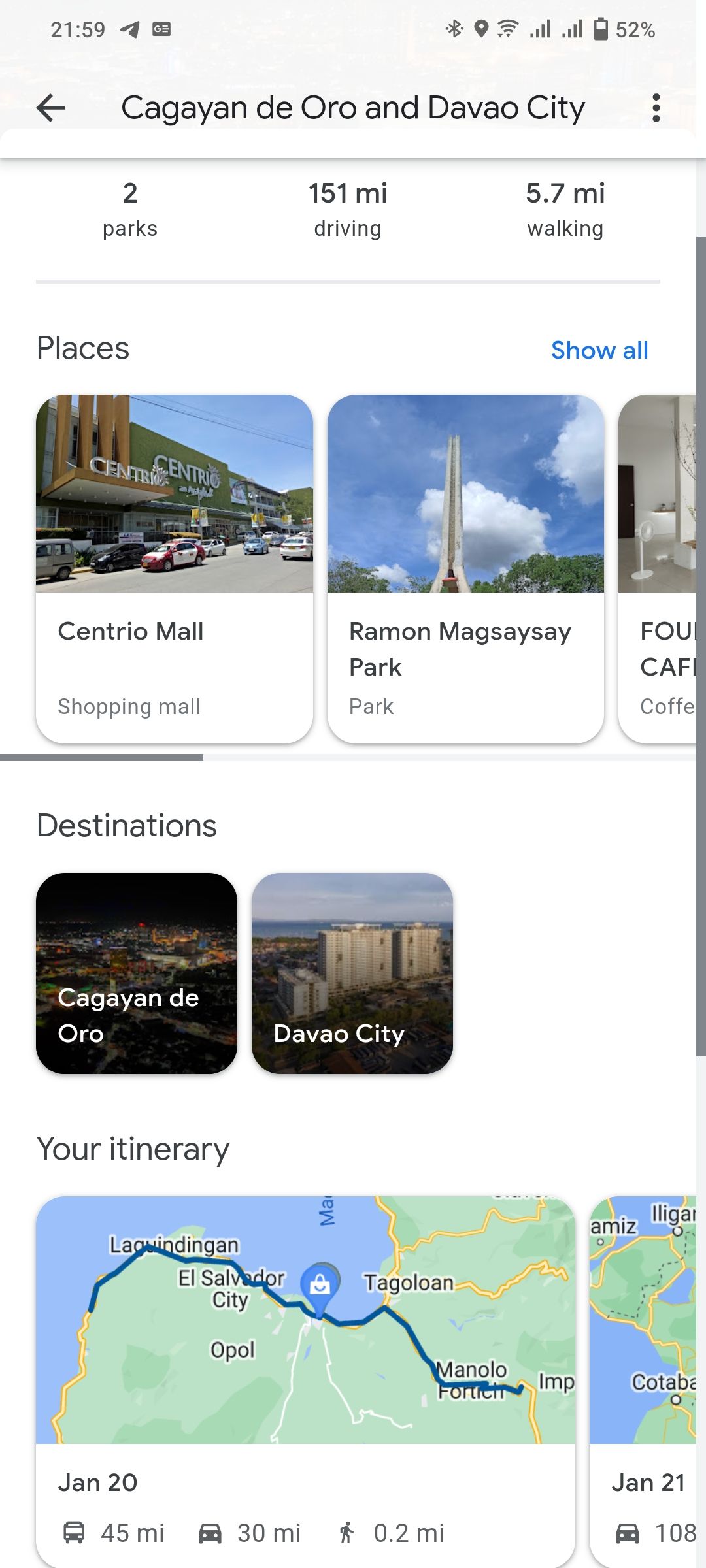This image captures a series of screenshots from a mobile device, showcasing a variety of informational elements and user interface icons. In the top-left corner, the time is displayed as 21:59, indicating it is 9:59 PM. Moving to the top-right corner, several icons are visible: a Bluetooth connected icon, an active location icon, a Wi-Fi signal icon, network signal bars for two SIM cards (SIM1 and SIM2), and a battery level indicator showing 52% charge remaining.

Within the search field, the user has entered "Kegeyan de Oro" and "Davao City." The results shown include multiple transportation options and distances — 151 miles by driving and 5.7 miles by walking. Among the places listed are two parks and several other points of interest like shopping malls and Ramon Magsaysay Park. There is also mention of destinations, including but not limited to Kegeyan de Oro and Davao City, forming part of an itinerary. The screenshot features names of various cities and locations, including Tegoluan and Opor, potentially as part of the planned route or points of interest along the way. The interface gives a comprehensive overview of geographic and navigational details pertinent to the selected destinations.